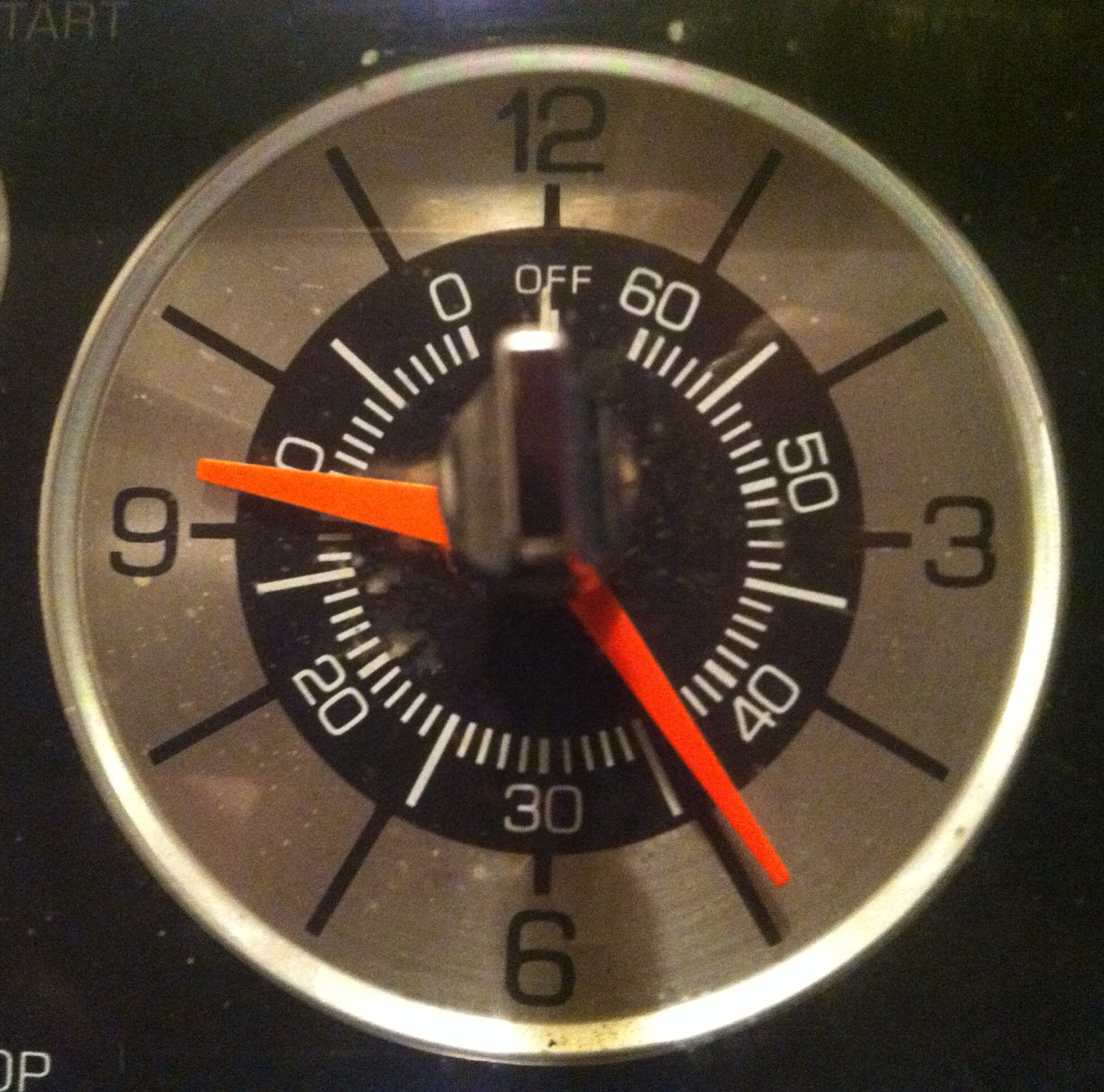The image is a close-up photograph of a chrome circular clock, possibly part of a stove or timer. The clock, set against a pure black background, prominently features large black numerals at 12, 3, 6, and 9 positions, forming a traditional clock face. The hour and minute hands are both red, adding a vivid contrast against the metallic surface. There is no second hand. Centrally located within the clock is a minute timer, currently set to the 'off' position. This timer displays markings for 60, 50, 40, 30, 20, 10, and 0, allowing for precise time setting in a circular arrangement. Small white dots indicate the seconds. The entire image emphasizes the functional and sleek aesthetic of the clock.